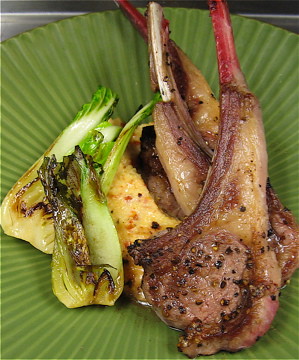The close-up image captures a vivid and detailed culinary scene. At the center of attention is a circular, frilly-edged green porcelain plate with distinct grooves along its rim. The plate hosts a modest assortment of food items, each presented with care. 

On the right side of the plate, two succulent chicken legs, expertly grilled and seasoned, exhibit a subtle char at the ends of their drums. Interestingly, these were initially thought to be lamb or a type of beef steak, indicating the rich, fatty texture and bone-in construction adding to the meaty indulgence.

On the left side, a bed of grilled greens, likely bok choy, showcases a delicate, slightly burnt edge. Tucked beneath these greens, flatter pieces of chicken breast reveal themselves, adding to the dish’s variety.

Underneath the grilled greens, a mysterious yellowish, spongy item hints at what could be a sauce or egg, adding an intriguing element to the presentation. The convergence of these textures and flavors on the beautifully adorned green plate creates a visually appealing and appetizing scene.